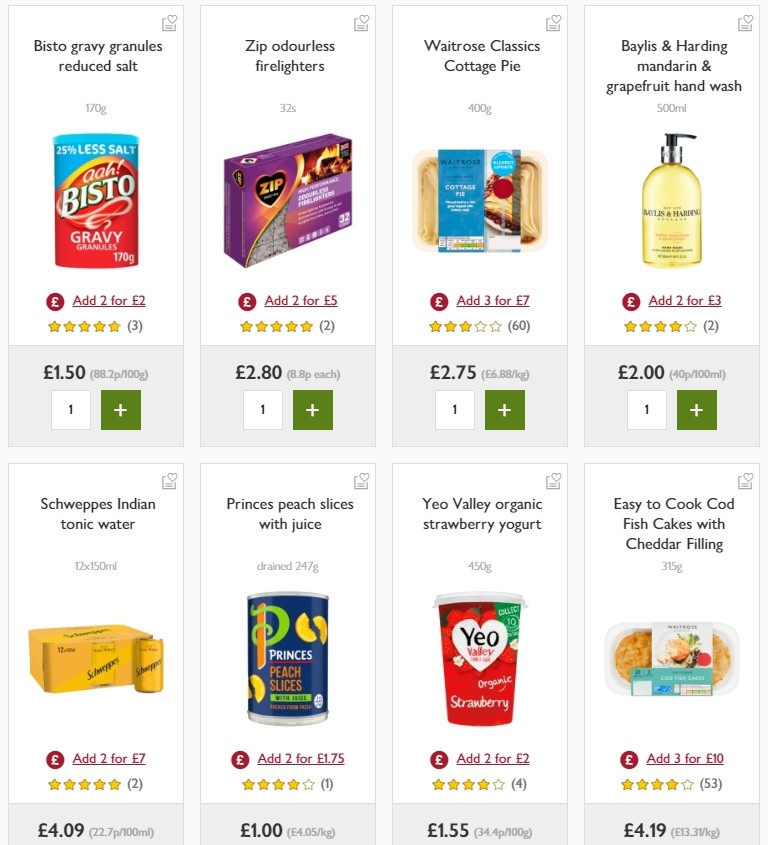This screenshot from an unspecified source showcases various items available for sale, complete with images, prices, discounts, and customer ratings. The detailed information provided is as follows:

1. **Bisto Reduced Salt Gravy Granules, 170g**
   - **Image:** Blue and red canister
   - **Description:** "25% less salt" in bold letters, with the brand-name "Ah! Bisto"
   - **Offer:** Add 2 for £2.00
   - **Rating:** 5 stars based on 3 reviews
   - **Price:** £1.50 (88.2p per 100g)
   - **Quantity:** 1

2. **Zip Odorless Firelighters, 32 pieces**
   - **Image:** Box of firelighters
   - **Offer:** Add 2 for £5.00
   - **Rating:** 5 stars based on 2 reviews
   - **Price:** £2.80 (8.8p each)
   - **Selected Quantity:** 1

3. **Waitrose Classics Cottage Pie, 400g**
   - **Image:** Package of cottage pie
   - **Offer:** Add 3 for £7.00
   - **Rating:** 3 stars based on 60 reviews
   - **Price:** £2.75 (6.88 per kg)
   - **Selected Quantity:** 1

4. **Baylis & Harding Mandarin and Grapefruit Hand Wash, 500ml**
   - **Image:** Yellow bottle with a black pump dispenser
   - **Offer:** Add 2 for £3.00
   - **Rating:** 4 stars based on 2 reviews
   - **Price:** £2.40 (48p per 100ml)
   - **Selected Quantity:** 1

5. **Schweppes Indian Tonic Water, 12 x 150ml**
   - **Image:** Orange carton and can of Schweppes
   - **Offer:** Add 2 for £7.00
   - **Rating:** 5 stars based on 2 reviews
   - **Price:** £4.09 (22.7p per 100ml)

6. **Princes Peach Slices with Juice (Drained), 247g**
   - **Image:** Blue can of peaches
   - **Offer:** Add 2 for £1.75
   - **Rating:** 4 stars based on 1 review
   - **Price:** £1.00 (405p per kg)

7. **Yeo Valley Organic Strawberry Yogurt, 450g**
   - **Image:** Container of yogurt
   - **Offer:** Add 2 for £2.00
   - **Rating:** 4 stars based on 4 reviews
   - **Price:** £1.55 (34.4p per 100g)

8. **Easy to Cook Cod Fish Cakes with Cheddar Filling, 315g**
   - **Image:** Packaged fish cakes
   - **Offer:** Add 3 for £10.00
   - **Rating:** 4 stars based on 53 reviews
   - **Price:** £4.19 (13.31 per kg)